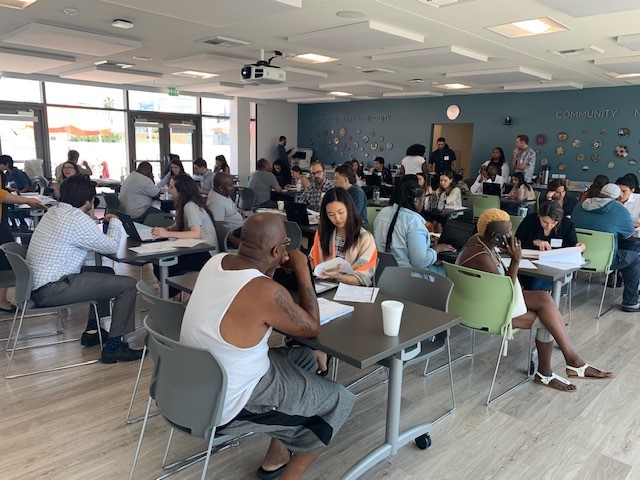The photograph captures a bustling, diverse room filled with people seated at rectangular black tables and dark gray and green plastic chairs. The setting resembles a cafeteria, with fluorescent ceiling lights casting a subdued glow over the grayish-beige wooden floors. A wide array of individuals—comprising African-Americans, white people, Asians, males, females, and varying ages—are engaged with documents and books, their expressions mostly serious. Some are dressed casually in shorts and tank tops, while others sport business casual attire. The room features prominent architectural details, including a wall completely covered in windows flooding the space with natural light, a dark blue back wall with an entryway, and a blue front wall with the word "community" visible. Additionally, a projector hangs from the ceiling, and there is an open door on one side. A notable figure in the scene is an African man on the right, while a woman in white sandals stands out in the foreground.